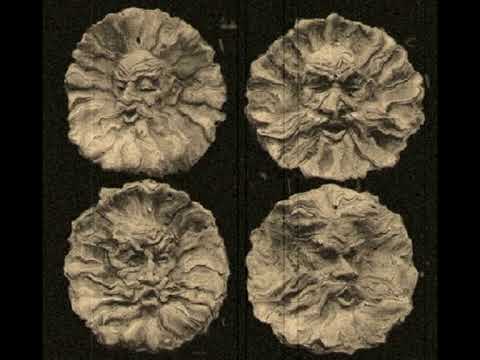The image consists of four distinct, circular clay sculptures mounted on a black background, each depicting the face of an old man with an emphasis on their mouths and wrinkles. The sculptures are a very light yellow with black stains, giving them a weathered, historical appearance. These plaques resemble a depiction of celestial bodies like the sun or moon, with wavy rays that radiate outward and integrate with the facial features, such as the beards and mustaches of the men.

- The top left face is turned to the left, with closed eyes and an open mouth, featuring prominent forehead wrinkles and a design incorporating the beard into the circle.
- The top right face looks straight ahead, with dark shadows over the eyes, a forward-thrusting mouth with a black interior, and a thick goatee mustache spreading sideways.
- The bottom left face is turned to the right, with open eyes (the left one wider), a slightly open mouth, and a circular pattern of wrinkles.
- The bottom right face has its head turned further right, with shadows over the eyes, a slightly open parched mouth, a large nose, and several streaks descending from the nose.

The black and white image is grainy and scratched, suggesting it might be a still from an old silent film, adding an ancient, timeless quality to the overall depiction.